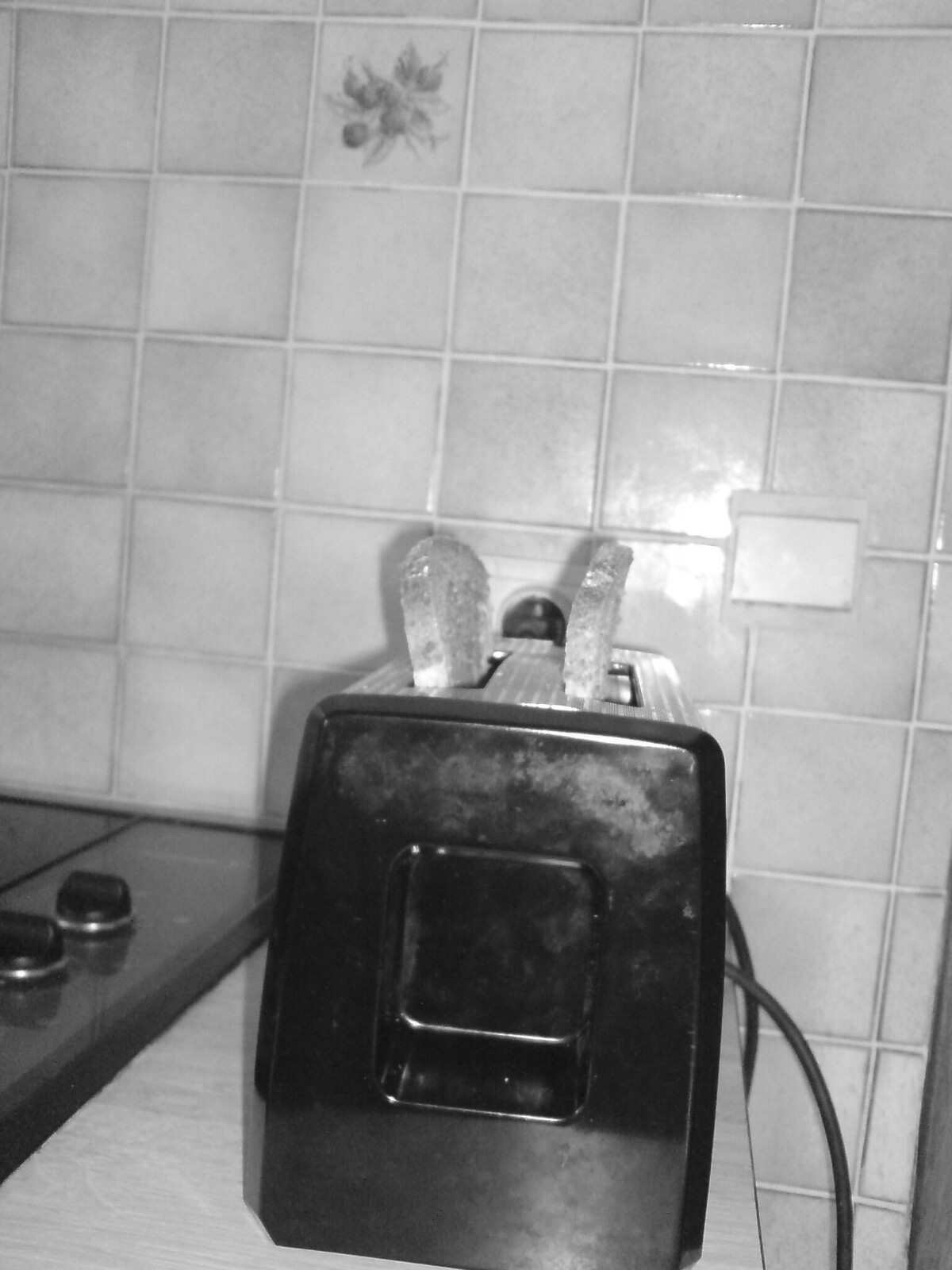This black and white photograph captures a nostalgic kitchen scene featuring an older-style black toaster with a metal frame, sitting on a light-colored counter. Emerging from the toaster are two pieces of bread, halfway out, appearing toasted. The counter, potentially marble or light stone, extends to an electric stovetop with two visible knobs to the left of the toaster. In the background, a wall tiled with square ceramic tiles adds texture; one of the tiles showcases a floral decal, possibly roses. The grayscale palette reveals fingerprint smudges on the toaster's front. Additionally, a light switch is noticeable on the right side of the image, near the electrical plug-in cord of the toaster, adding to the detailed domestic setting.